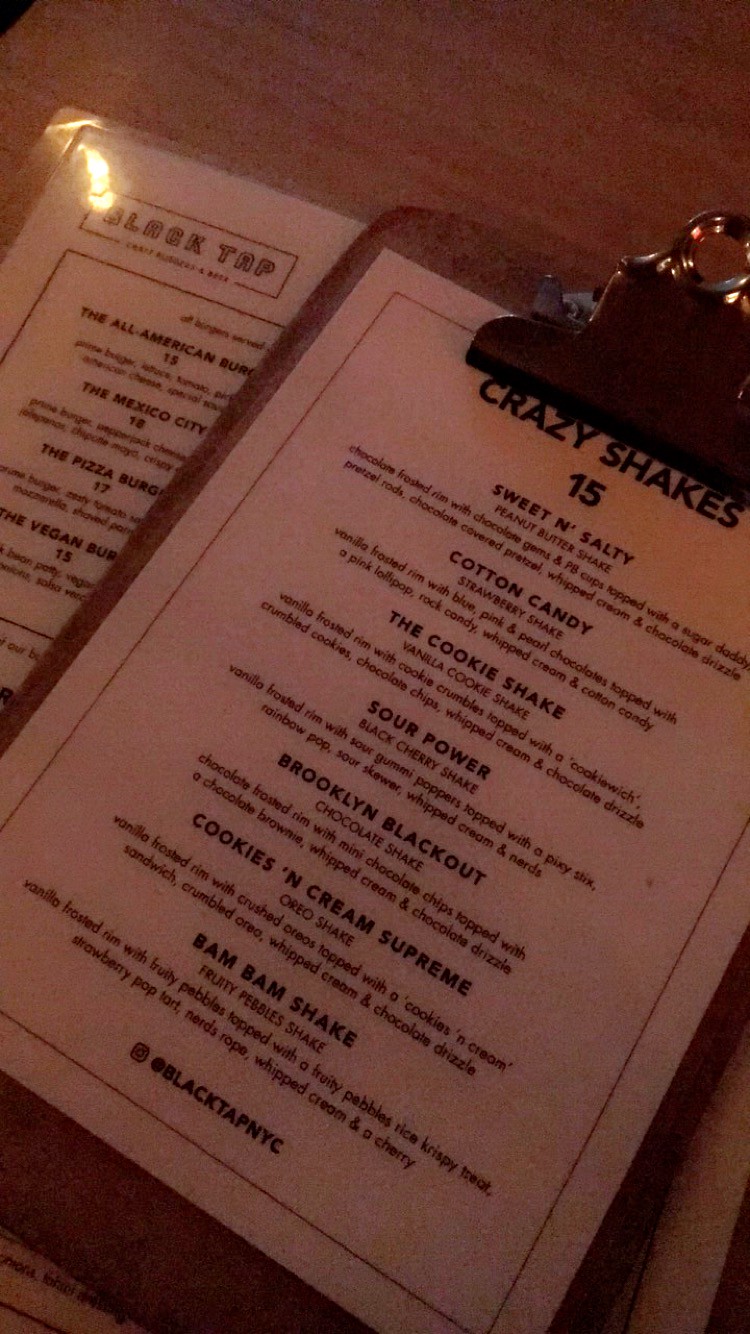This is a detailed aerial photograph featuring a vintage-style clipboard made from brown cork, complete with a brown clip and a silver ring at the top. The clipboard holds a vertically rectangular laminated menu that's white with a faint black outline. At the top, "Crazy Shakes" is prominently displayed in black, font size 15, followed by a list of intricately described shakes. The shakes included are:

1. **Sweet and Salty**
2. **Cotton Candy**
3. **The Cookie Shake**
4. **Sour Power**
5. **Brooklyn Blackout**
6. **Cookies and Cream Supreme**
7. **Bam Bam Shake**

Each shake name is followed by a detailed ingredient list. At the very bottom, a copyright notice reads, "Black Tap New York City."

The clipboard is placed at an angle, revealing a second menu beneath it on the brown wooden table. This secondary menu has "Black Tap" prominently at the top left corner, followed by a food menu listing various burger options such as the All-American Burger, the Pizza Burger, and the Vegan Burger, each with corresponding prices. The overall setup suggests a rustic yet modern dining ambiance.